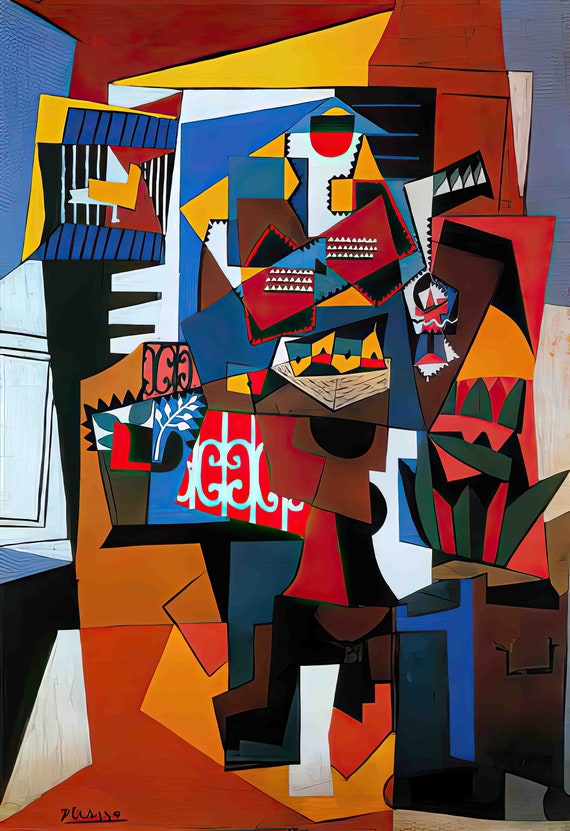This painting by Pablo Picasso is a striking example of his cubist and abstract work. It features a vividly colorful composition characterized by geometric shapes such as squares, triangles, and circular forms. The palette includes bold reds, blues, yellows, oranges, whites, and dark greens, creating a visually dynamic scene. The elements are distinctly blocky and chunky, arranged in a seemingly chaotic manner that is typical of collage-style art. Key features include a blue block with black stripes, a black square with white stripes, gold triangles, and a piece that resembles folded paper. Though abstract and not immediately decipherable, the artwork hints at figures and objects like a piano and possibly a creature with a beak. The background appears white, setting off the intricate, vibrant patterns that give the painting its dynamic and jumbled feel.